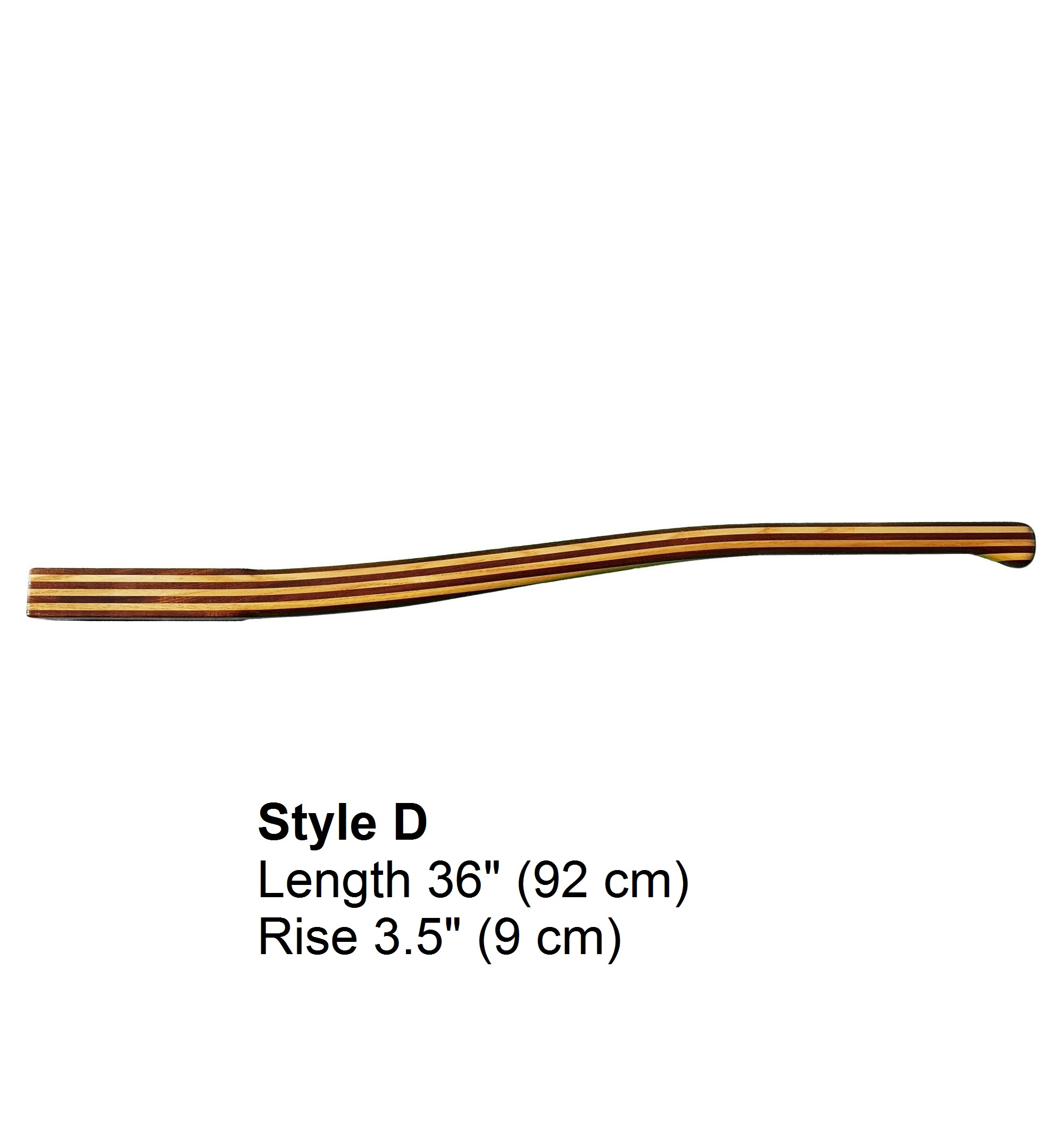The image features a laminated wooden item, likely a guitar neck, displayed against a completely white background. The object is composed of several alternating layers of dark brownish-reddish wood and light-colored wood, creating a striped pattern. The lamination alternates with layers in the sequence: dark, light, dark, light, and so on. The thickness of the piece varies along its length—it starts thicker at one end, curves, tapers thinner in the middle, and then thickens slightly at the other end. Below the item, in black type, the following text is displayed: "Style D, Length 36 inches (92 centimeters), Rise 3.5 inches (9 centimeters)."